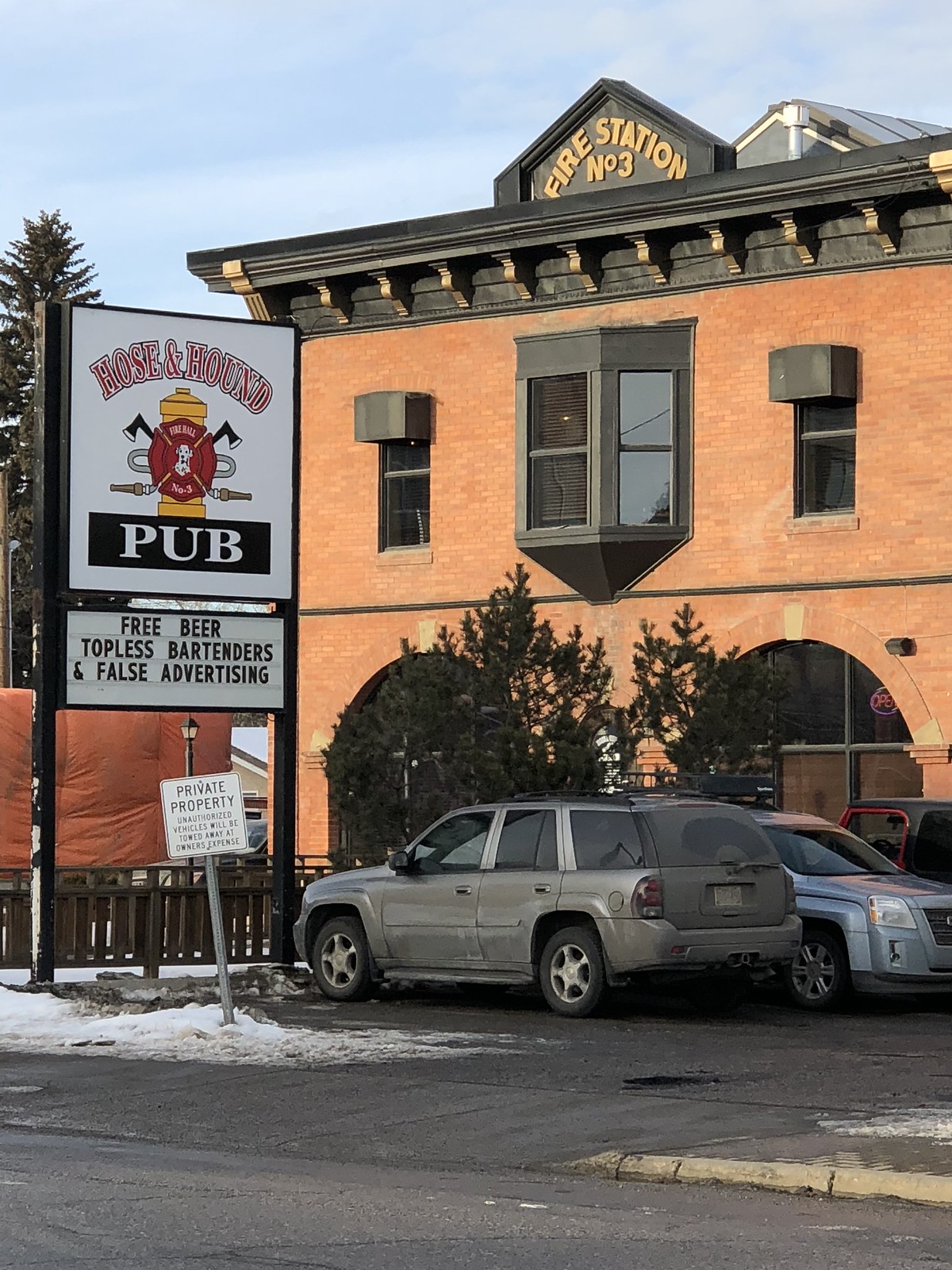This detailed, full-color photograph taken outdoors during the day captures a converted fire station that now serves as a pub named "Hose and Hound Pub." The building is made of orange brick and features a distinct roofline with a sign at the top that reads "Fire Station Number Three." The second floor has three windows, with one being a prominent bay window. Below the windows, the building has two large archways, flanked by trees. A tall pine tree stands to the far left of the structure.

In front of the building, there is a parking lot with a yellow curb and ramp leading onto it. Two cars, a silver sedan and a grey station wagon, are parked in the lot. The scene is enhanced by a clear sky with light clouds.

Mounted on the building is a cheeky sign that reads "Hose and Hound Pub" with a fire hydrant and firefighter emblem logo, and below it, messages that playfully state: "Free Beer, Topless Bartenders, and False Advertising." Beneath this sign is another sign that reads "Private Property, Unauthorized Vehicles Will Be Towed Away at Owner's Expense."

Overall, this image strikingly combines the historical architecture of a fire station with the vibrant, whimsical charm of a modern pub.